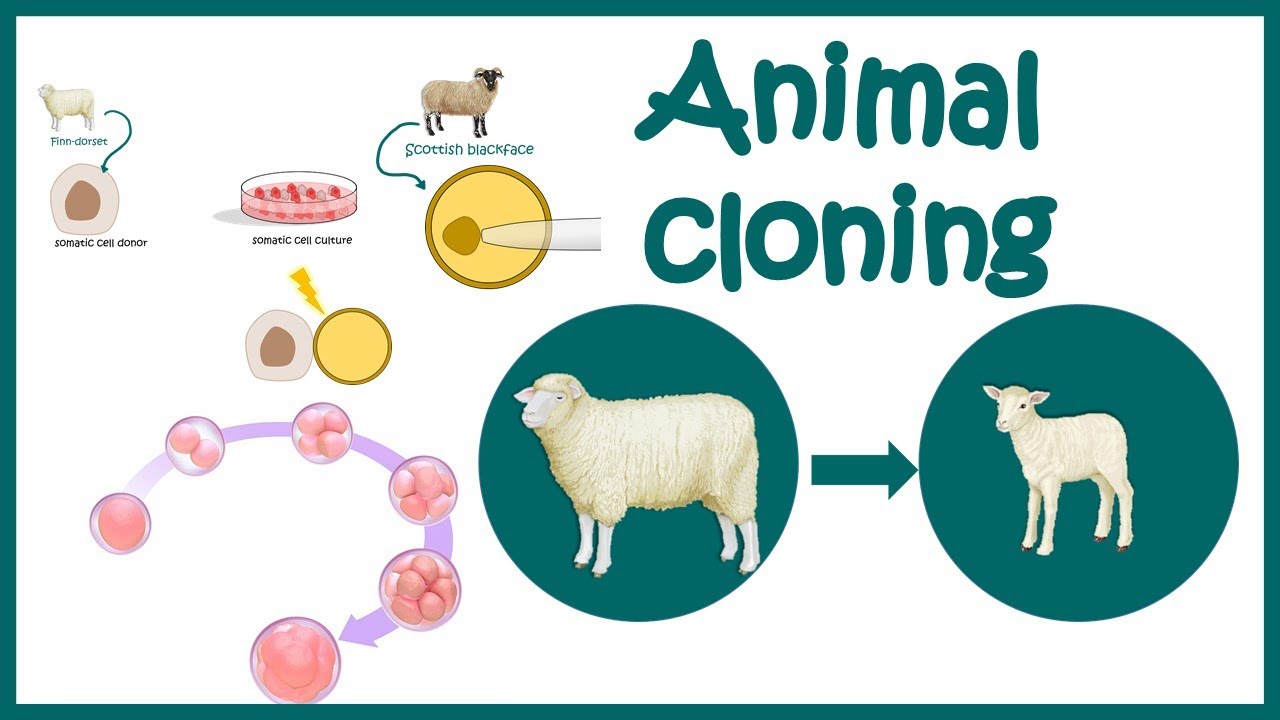The infographic poster titled "Animal Cloning," bordered in dark green, aims to explain the cloning process. Dominated by two large teal circles on the right, it features an adult Finn Dorset sheep in the left circle with an arrow pointing towards a lamb in the right circle, suggesting the cloning result. The top of the poster labels a small lamb as "Scottish Blackface." On the left side, detailed cartoon drawings illustrate various stages of cell division and injection of DNA material into cells. There's a depiction of a petri dish labeled "somatic cell culture" and multiple images of cells to elaborate the cloning procedure. Despite its informative intent, the poster's clarity on the cloning process is somewhat lacking.